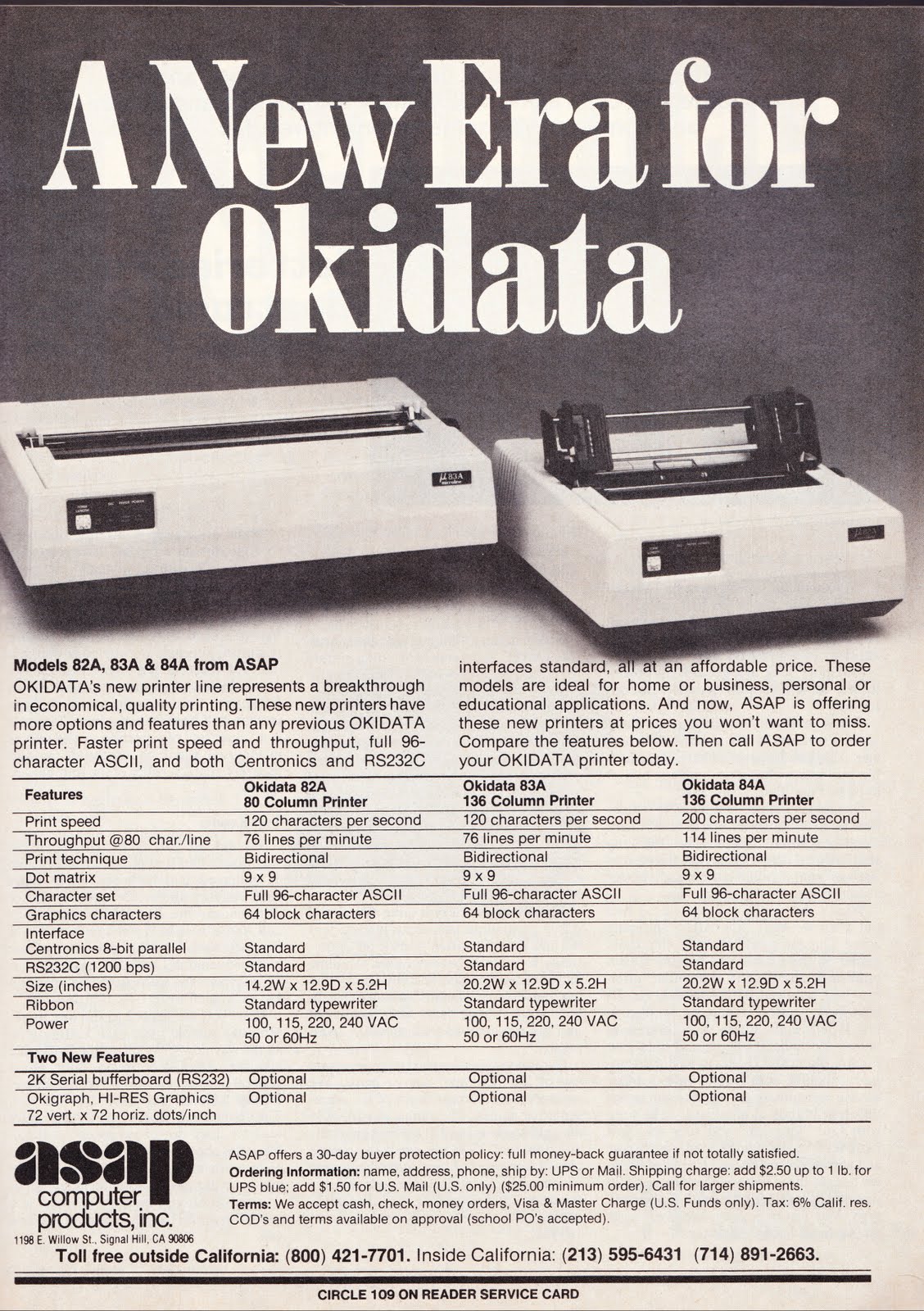This rectangular, vintage advertisement, approximately six inches tall and four inches wide, seems to be a page taken from an old newspaper or magazine with an aged off-white, almost brownish tone. It predominantly features grayscale shades. The top third of the ad has a dark gray, almost black background with large, bold white text declaring, "A New Era for Okidata."

Below this headline, there are black and white photos of two white computer printers side-by-side; the printer on the right has a paper holder standing upright. Following the images is detailed, bold black text introducing the models 82A, 83A, and 84A from ASAP Computer Products, Inc. The adjacent description comprises two paragraphs elaborating on the features of the Okidata printers.

Underneath the descriptive text, there's a grid or table comparing the specifications for each printer model. The table outlines key features such as print speed, throughput, print technique (dot matrix), character set, graphics capabilities, interface specifics (8-bit parallel), power requirements, and optional features.

At the bottom left corner, the advertisement provides the company’s name, ASAP Computer Products, Inc., along with various contact details: a toll-free number for calls outside California (800-421-7701) and local numbers for calls within California (213-595-6431 or 714-891-2663). A thin black horizontal line spans from left to right at the bottom of the image, and beneath it, the text instructs, “circle 109 on reader service card.”